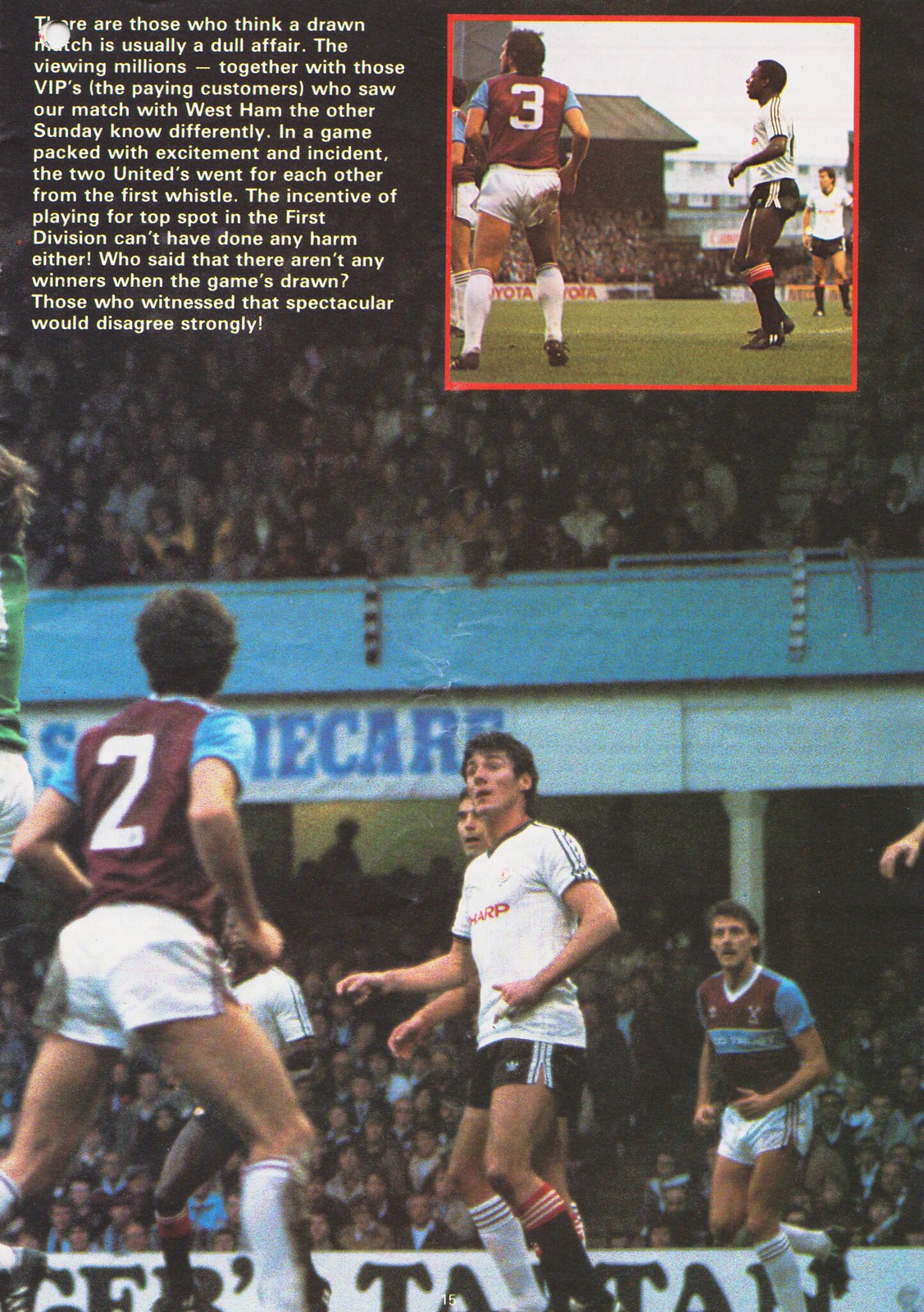This image, appearing to be a page from a British football (soccer) magazine or program, features a detailed and dynamic scene from a professional soccer match. In the top right corner, a prominent photograph showcases five players actively engaged in the game. One team is dressed in white shirts with black shorts, while the opposing team sports maroon shirts with white shorts. Among the maroon team players, number two stands out as he gazes towards the crowd, adding a narrative depth to the scene.

In the background, the image vividly captures the bustling atmosphere of the stadium. Hundreds of fans fill the stands, which consist of an upper deck with a blue railing and a lower deck with a white railing, both packed to capacity. The upper left corner of the page features text overlaying the image, partially covering the sponsorship names visible along the stands. 

The text reads, "There are those who think a drawn match is usually a dull affair. The viewing millions, together with those VIPs, the paying customers who saw our match with West Ham the other Sunday, know differently. In a game packed with excitement and incident, the two Uniteds went at each other from the very first whistle. The incentive of playing for top spot in the First Division can't have done any harm, either. Who said there aren't any winners when the game is a draw? Those who witnessed that spectacle would agree strongly."

Additionally, there is a smaller inset image providing a different view of the stands, giving the entire scene a layered, multimedia feel. The layout includes an orange border around the primary photo, contributing to the visual structure of the page. The overall tone of the image and text emphasizes the excitement and competitive spirit of the match, highlighting the vibrant fan presence and the significance of the game’s draw.